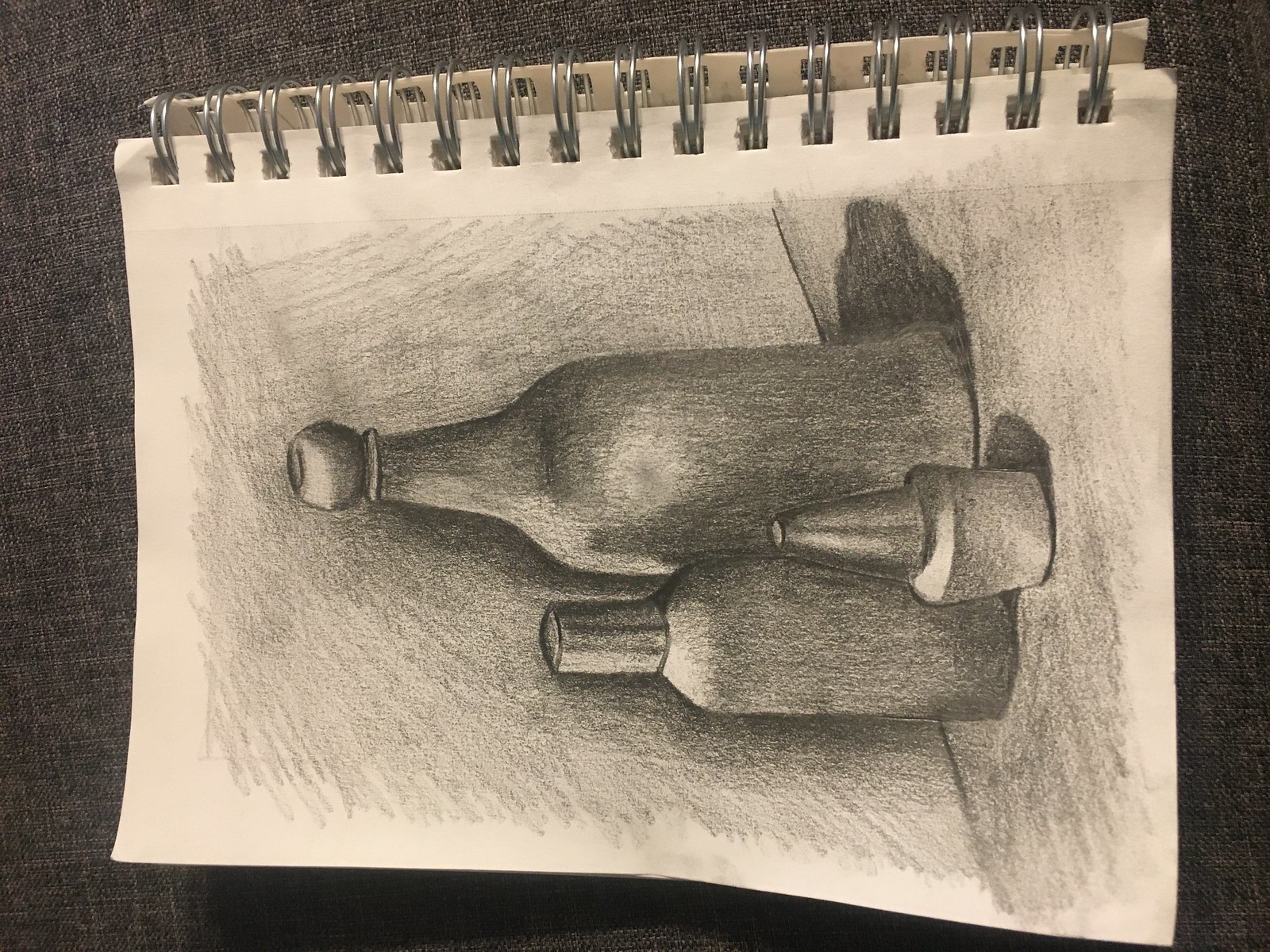This pencil drawing, rendered with meticulous shading, depicts three distinct bottles, each uniquely shaped and topped. The smallest bottle resembles a nail polish container, featuring an abbreviated cone-shaped top. The medium-sized bottle appears to be a spray bottle with a cylindrical lid. The tallest bottle boasts a spherical cap, adding to the diversity of forms. All three bottles rest on a flat surface, likely a table, meticulously shaded to convey dimension. Behind them, a textured wall provides a backdrop, also richly shaded to enhance the scene's depth. This detailed sketch is part of a spiral-bound sketchbook, which lies on a table draped with a brown tablecloth, subtly grounding the artwork in a realistic setting.